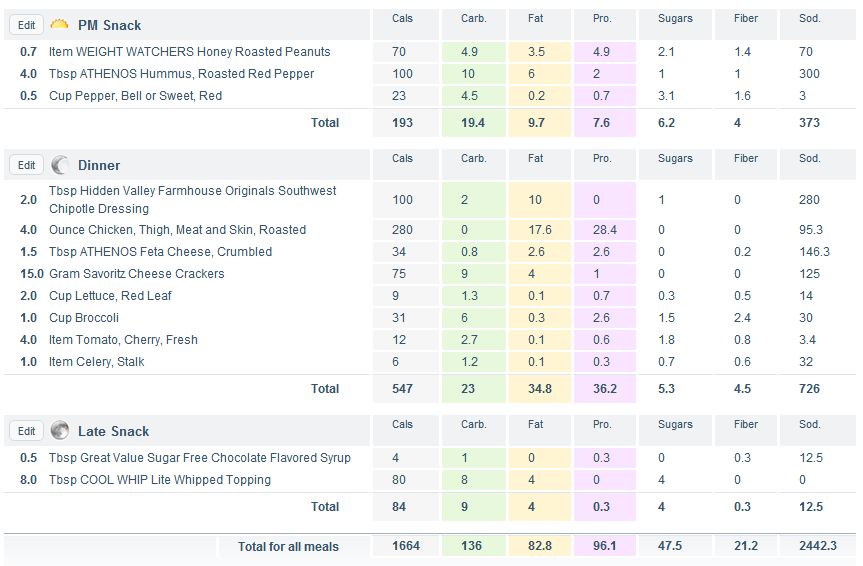This detailed chart highlights the nutritional breakdown of a p.m. snack, dinner, and a late snack. The information is presented in blue letters on a white background, with each meal meticulously analyzed in terms of calories, carbs, fat, protein, sugars, fiber, and sodium.

**P.M. Snack:**
- **Weight Watchers Honey Roasted Peanuts:** 70 calories, 4.9g carbs, 3.5g fat, 4.9g protein, 2.1g sugars, 1.4g fiber, 70mg sodium.
- **Athenos Hummus (Roasted Red Pepper, 4 tablespoons):** 100 calories, 10g carbs, 6g fat, 2g protein, 1g sugars, 1g fiber, 300mg sodium.
- **Half a cup of Red Bell Pepper:** 23 calories, 4.5g carbs, 0.2g fat, 0.7g protein, 3.1g sugars, 1.6g fiber, 3mg sodium.

*Total for P.M. Snack:* 193 calories, 19.4g carbs, 9.7g fat, 7.6g protein, 6.2g sugars, 4g fiber, 373mg sodium.

**Dinner:**
- **Hidden Valley Farmhouse Southwest Chipotle Dressing (2 tablespoons):** 100 calories.
- **Chicken Thigh (Meat and Skin, Roasted, 4.0 ounces):** 280 calories.
- **Athenos Feta Cheese (1.5 tablespoons):** 34 calories.
- **Savoritz Cheese Crackers (15 grams):** 75 calories.
- **Red Leaf Lettuce (2 cups):** 9 calories.
- **Broccoli (1 cup):** 31 calories.
- **Cherry Tomatoes (4 pieces):** 12 calories.
- **Celery Stalk (1 piece):** 6 calories.

*Total for Dinner:* 547 calories.

**Late Snack:**
- **Great Value Sugar-Free Chocolate Flavored Syrup (0.5 tablespoons):** 4 calories.
- **Cool Whip Light Whip Topping (8 tablespoons):** 80 calories.

*Total for Late Snack:* 84 calories.

**Total for All Meals:**
- **Calories:** 1,664
- **Carbs:** 136g
- **Fat:** 82.8g
- **Protein:** 96.1g
- **Sugars:** 47.5g
- **Fiber:** 21.2g
- **Sodium:** 2,442mg